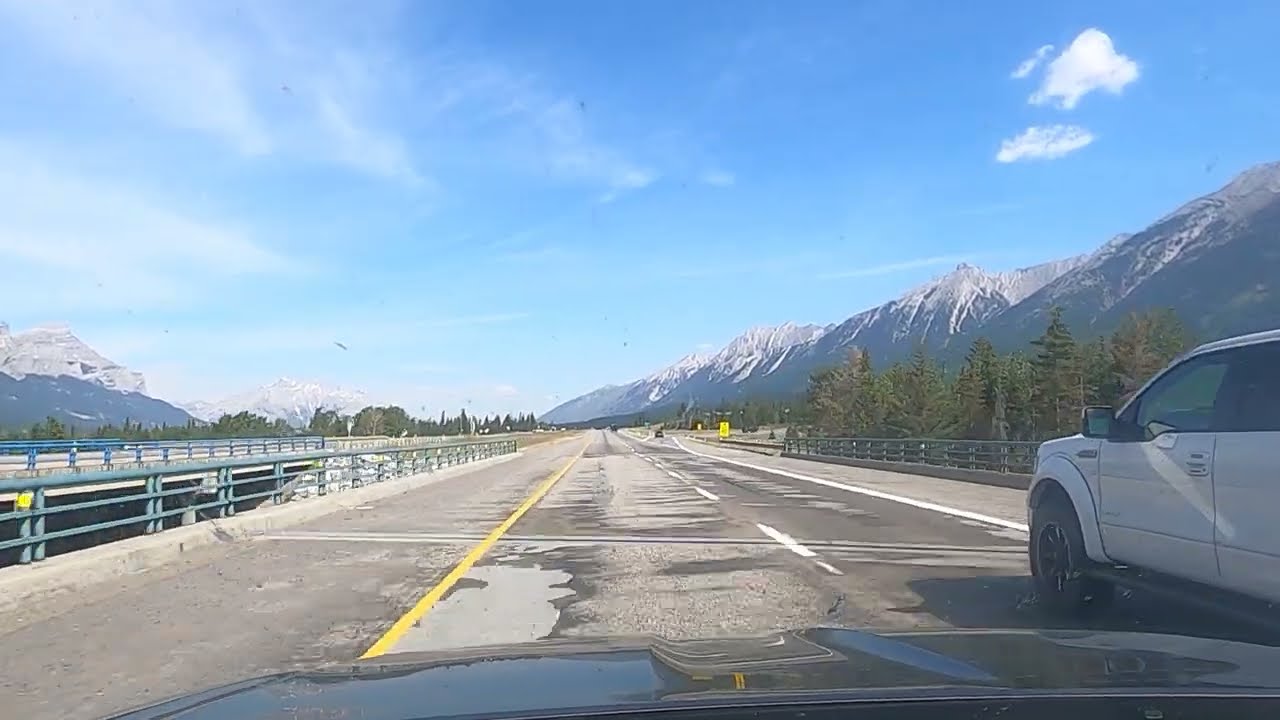This detailed photograph, captured from the driver's viewpoint of a black vehicle, showcases a long, paved highway set in a scenic mountainous landscape. The road, adorned with white dashed lines in the center, white lines on the right, and a yellow line on the left, stretches ahead beneath a bright blue sky dotted with hazy white clouds. The driver navigates a bridge with green metal railings, paralleled by another bridge for oncoming traffic on the left. To the right, a white pickup truck is visible slightly ahead, reflecting the road on its dark hood. Evergreen trees line the horizon, framing the majestic, snow-capped mountain range that spans both sides of the image. In the distance, the road splits into two directions beyond the bustling bridges, while birds soar above the picturesque scene.